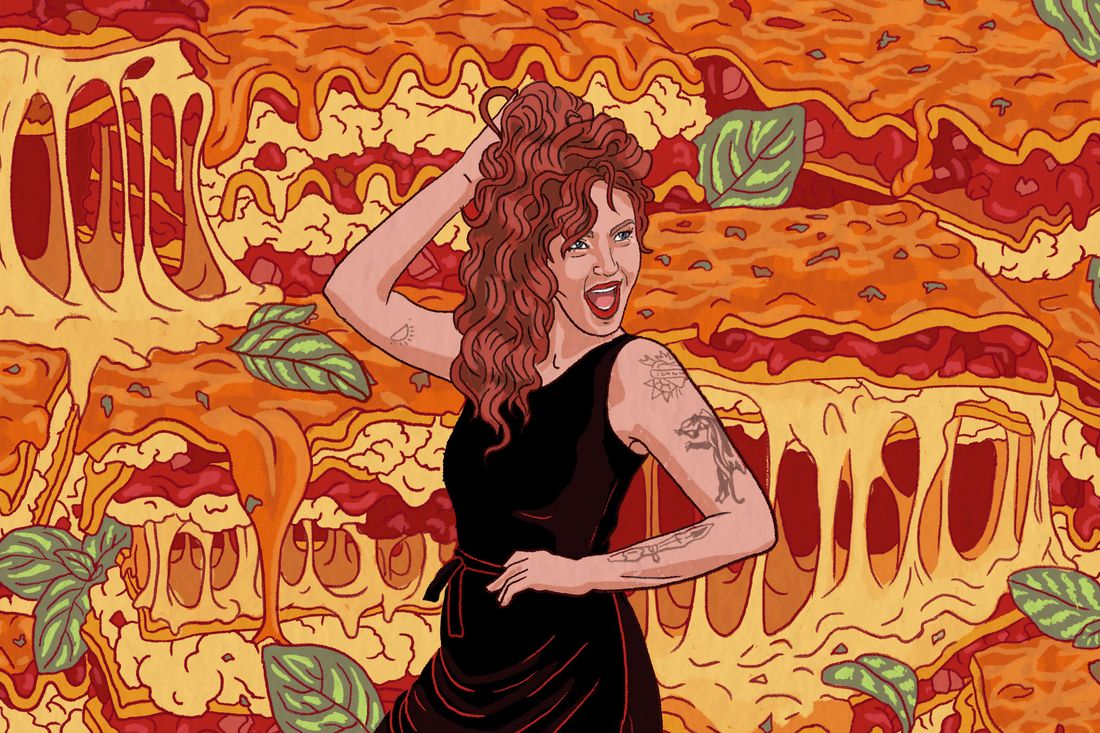The image is a vibrant, cartoon-style graphic featuring a lively female character who exudes energy and exuberance. She wears a dark, velvet-red, sleeveless dress with a ribbon tied around her waist. Her personality shines through her bright, blue eyes and expressive red lips, which she parts in an open-mouthed smile, revealing her teeth. The woman's long, curly hair is a distinctive shade of red and cascades freely down her back. Her left hand is raised to her hair, showcasing several intricate tattoos on her arms, including a heart, a paintbrush, a dragon, a sun, a cat, and an alligator. The backdrop is filled with detailed illustrations of lasagna, depicted with layers of noodles, red tomato sauce, white cheese, and green basil leaves, some pieces dripping with gooey, stringy cheese. The overall scene is dynamic and colorful, with the food elements adding a whimsical touch.